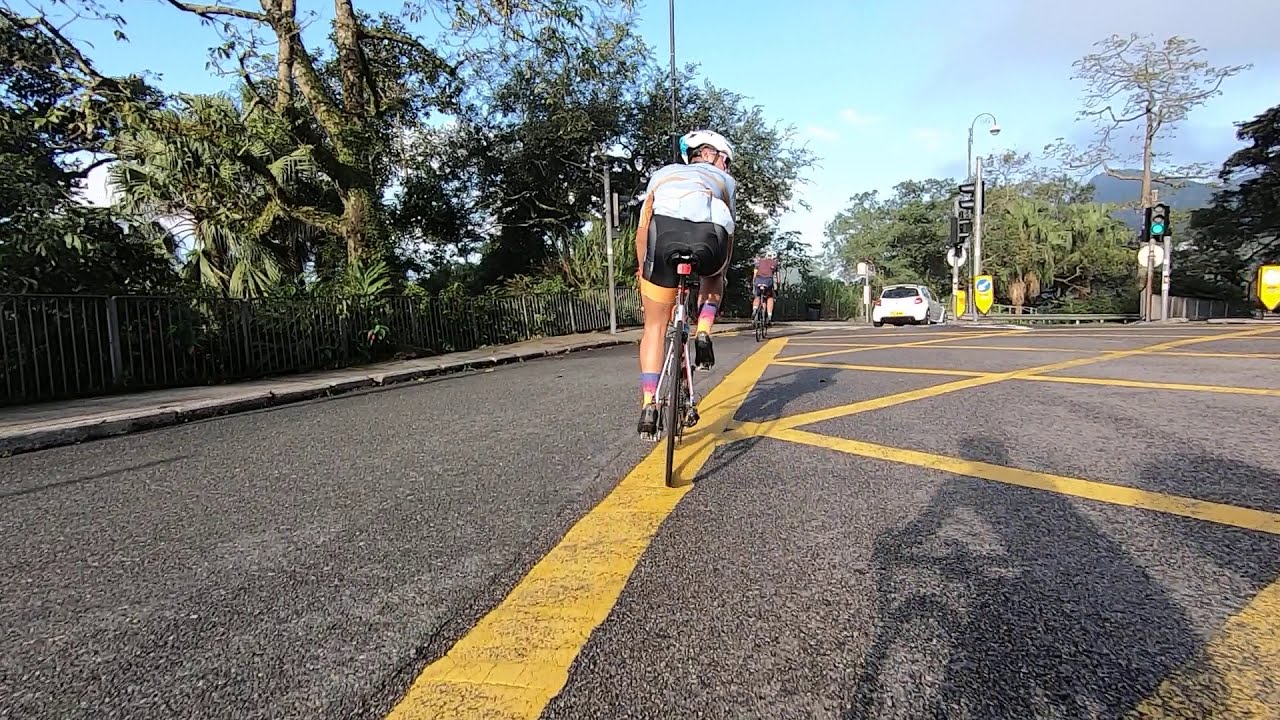This image captures a scene of three bicyclists riding on a wide section of an asphalt road. The photo appears to be taken from the perspective of the third bicyclist, as the shadows of the bike and rider are visible on the road. The foremost cyclist is wearing a white helmet, a white shirt, black pants, and rainbow-colored socks, while the second cyclist, slightly further ahead, is dressed in a purple shirt, black pants, and also a white helmet. In front of the cyclists, a white coupe car is visible, driving on the same road which features yellow diagonal lines indicating a crossing or an intersection, marked by a green traffic light.

To the left side of the road, there is a paved walk path bordered by a small fence, with tree trunks appearing beyond the fence, suggesting a steep drop-off or cliff edge. The background scenery includes lush trees and a mountain peak under a blue sky, scattered with light white clouds. On the right-hand side of the image stands a streetlight and a sign mounted on white pillars. The road appears to be curving sharply to the right, leading into a more wooded, country-like setting.